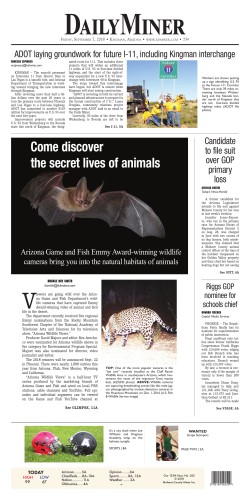Screenshot of the homepage of the Daily Miner, an online newspaper. The primary article features the Arizona Department of Transportation (ADOT) laying groundwork for the future Interstate 11, including the Kingman Interchange. Accompanying this article is an image of road crew workers installing a green freeway sign marked with "Interstate 11."

The second feature article is about bats, spotlighted by a striking image of a solitary bat flying against a black background. The image is captioned with white text that invites readers to "come discover the secret lives of animals."

Below the bat article is another photograph, this time of a leopard, indicating an article likely pertaining to wildlife or conservation.

On the right-hand side of the webpage, two smaller articles are listed: the first reports on a candidate intending to file a lawsuit over a GOP primary loss, and the second announces Riggs as the GOP nominee for school chief.

The bottom of the page includes various sections such as sports, featuring an update on football along with a scoreboard. A weather forecast for the day, displaying the expected high and low temperatures, is also present.

In the lower-right corner, there is a barcode and an image of a woman wearing a green tank top.